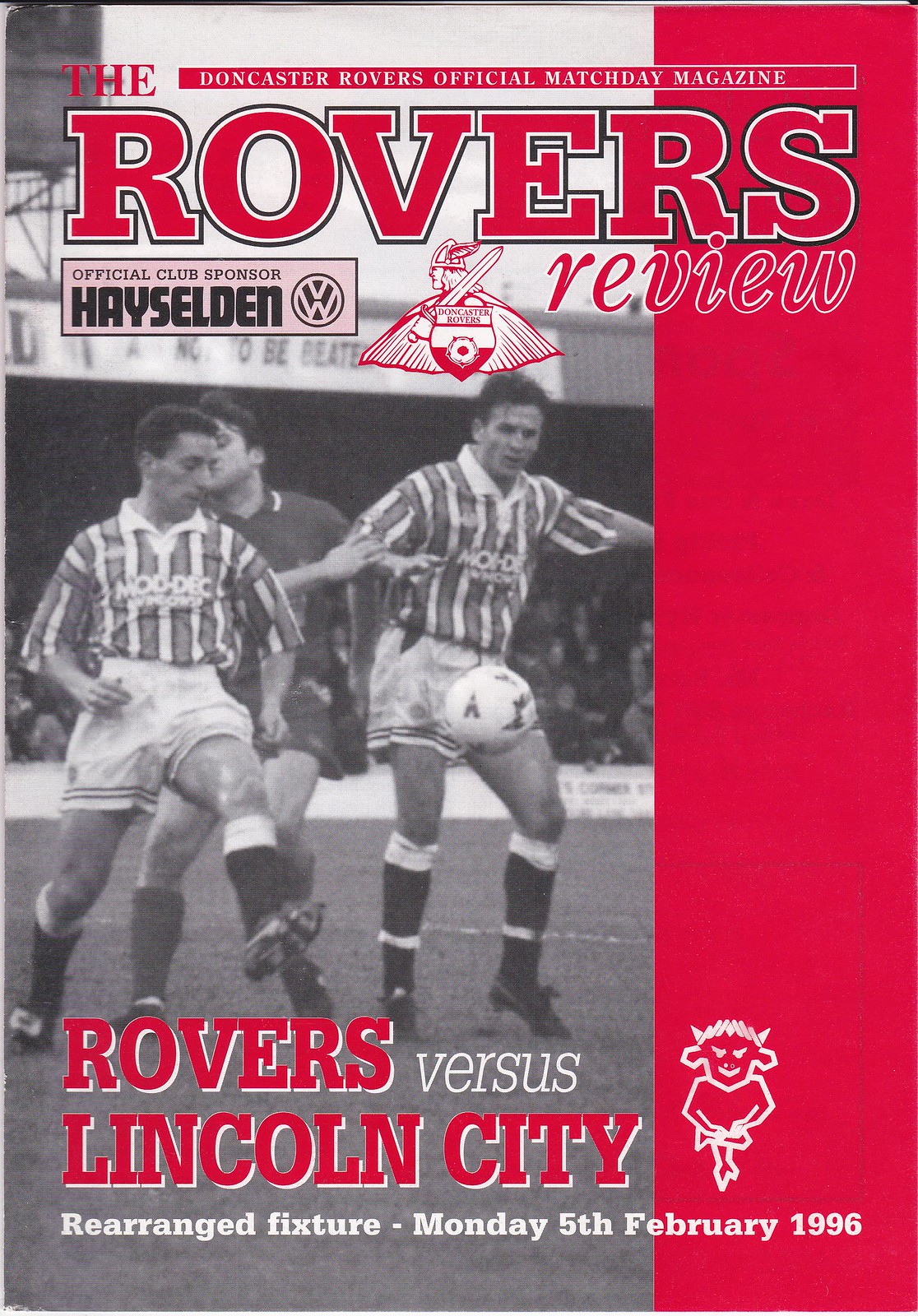The image is the front cover of a vintage soccer program dated Monday, 5th February 1996, for the rearranged fixture between the Rovers and Lincoln City. At the very top, red letters with black outline proclaim "The Rovers Review," with "Doncaster Rovers Official Match Day Magazine" printed in smaller letters just above it. Below this, in a pink rectangle, reads "Official Club Sponsor Hazelden." Towards the right is the Doncaster Rovers' logo, featuring a Viking with a sword, cape, and winged helmet. The main image covering the left three-quarters of the page is a black-and-white photo of two players in striped jerseys, seemingly in mid-action with a white ball in front of them, their legs extended and arms out. Another player in a solid-colored jersey is seen running towards them from the background, which shows the heads of spectators amidst a dark backdrop. A vertical red bar runs down the left side of the program. At the bottom, bold red letters announce "Rovers versus Lincoln City." All players are geared up in traditional soccer attire, including knee-high socks and cleats.